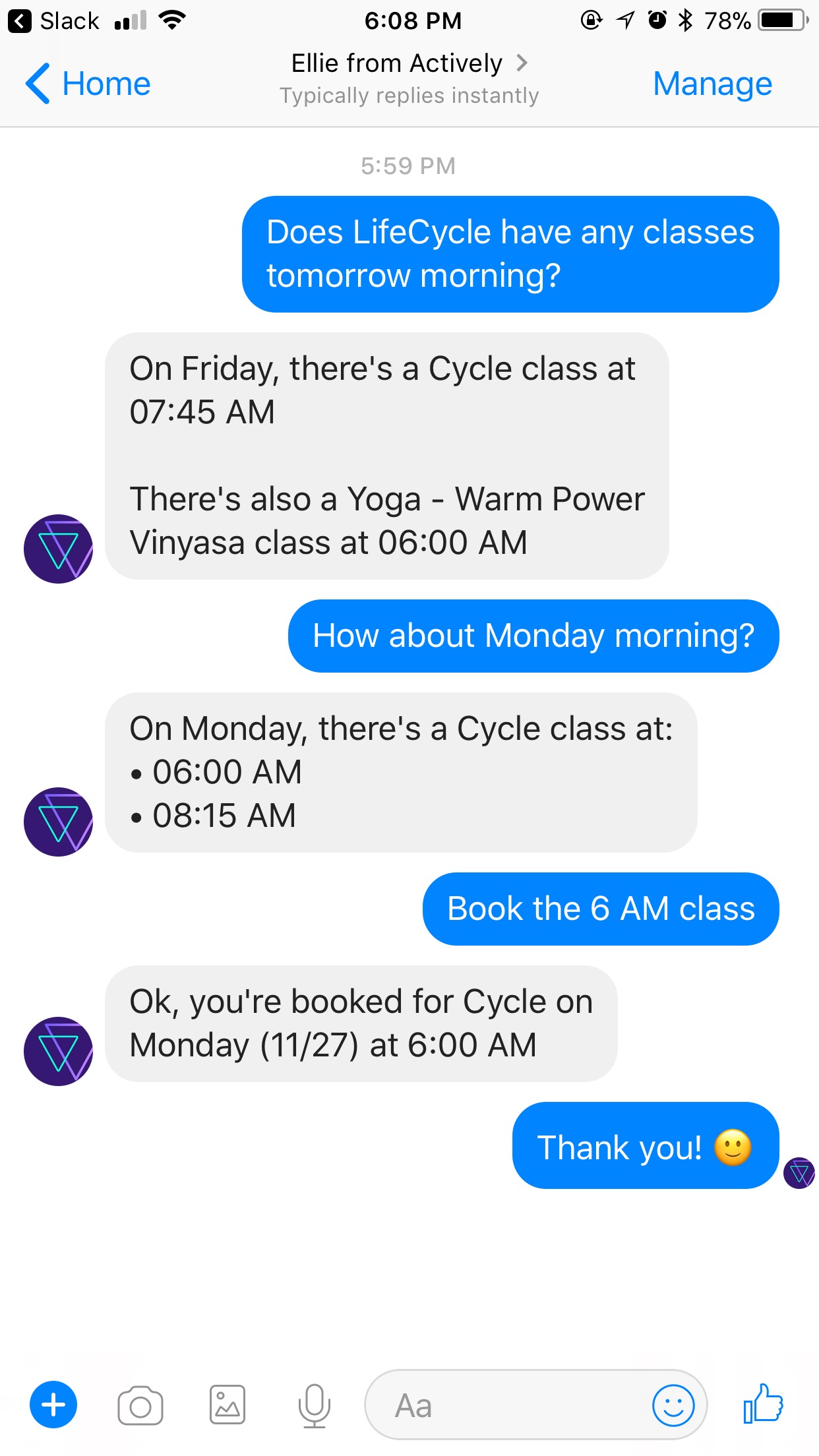Here is a detailed and cleaned-up caption:

---

A screenshot of a messaging app's chat thread, featuring an exchange between two individuals distinguished by their speech bubble colors—blue and light gray. The conversation begins with the person represented by blue text asking, “Does LifeCycle have any classes tomorrow morning?” The respondent in light gray replies, “On Friday, there is a cycle class at 7:45 a.m. and a yoga Vinyasa class at 6 a.m.” The person in blue follows up with, “How about Monday morning?” The response comes in light gray, “On Monday, there's a cycle class at 6 a.m. and another at 8:15 a.m.” The blue text then instructs, “Book the 6 a.m. class.” The person in gray confirms the booking, stating, “Okay, you’re booked for a cycle on Monday, 11/27 at 6 a.m.” The conversation concludes with the blue-texted individual expressing gratitude with, “Thank you :)”

---